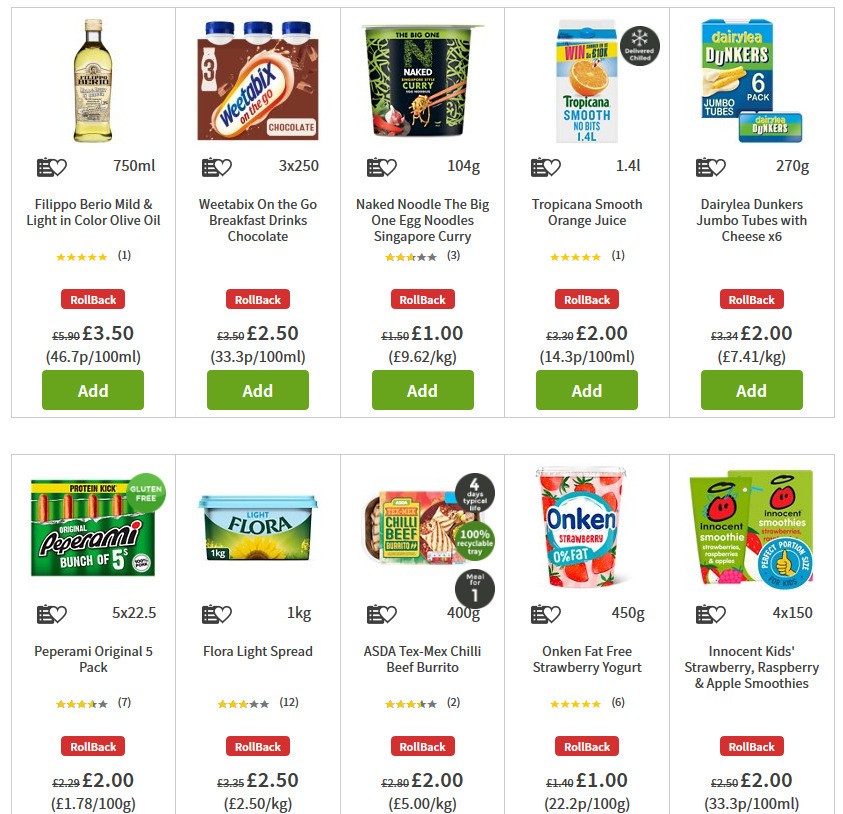This is a screenshot of a shopping page displaying ten different products arranged in two vertical sections, separated by a thin gray line and a white space in the middle. Each product is housed within its own section. From left to right, the products include:

1. Filippo Berio Mild & Light in Color Olive Oil.
2. Weetabix On-The-Go Breakfast Drinks Chocolate.
3. Naked Noodle The Big One Egg Noodles Singapore Curry.
4. Tropicana Smooth Orange Juice.
5. Dairylea Dunkers Jumbo Tubes with Cheese x6.
6. Pepperami Original 5-Pack.
7. Flora Light Spread.
8. ASDA Tex-Mex Chili Beef Burrito.
9. Onken Fat-Free Strawberry Yogurt.
10. Innocent Kids Strawberry, Raspberry, and Apple Smoothies.

Each product displays an image, followed by a star rating beneath it. Notably, Weetabix On-The-Go Breakfast Drinks, Innocent Kids Smoothies, and Dairylea Dunkers lack star ratings. Below each product image is a red "Rollback" button indicating a discount, and the price in GBP is listed beneath this button. The top row of products includes a green "Add" button for easy addition to the shopping cart, but the bottom row of products is partially cut off and does not show the "Add" button.